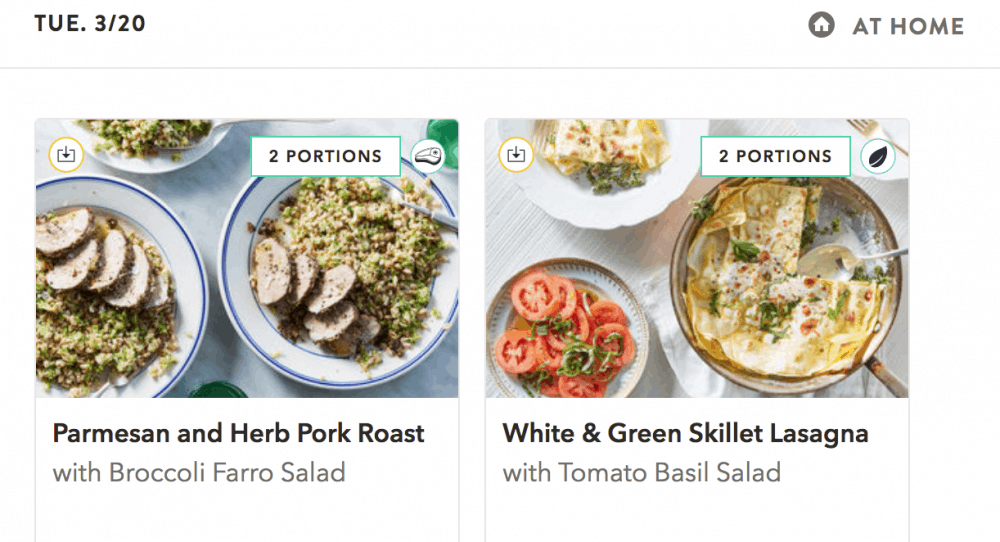The top left corner of the image displays the text "TUE. 3-20," indicating the date is Tuesday, March 20th. In the top right corner, there is a home icon accompanied by the text "at home." 

At the bottom of the image, there are two side-by-side photographs of meals. 

The left photograph features a recipe for "Parmesan and Herb Pork Roast with Broccoli Farro Salad." Displayed are two plates containing the dish, each with approximately five slices of pork roast. Visible on the plates are vibrant bits of broccoli and grains of farro, all garnished with a sprinkling of parmesan cheese. A rectangular box within this section states "two portions" and includes options, likely for downloading or sharing the recipe.

The right photograph showcases a recipe for "White and Green Skillet Lasagna with Tomato Basil Salad." The lasagna is served in a skillet, highlighting its white and green layers. Alongside, there's a plate with sliced tomatoes topped with fresh basil. This section also notes that the dish serves two portions.